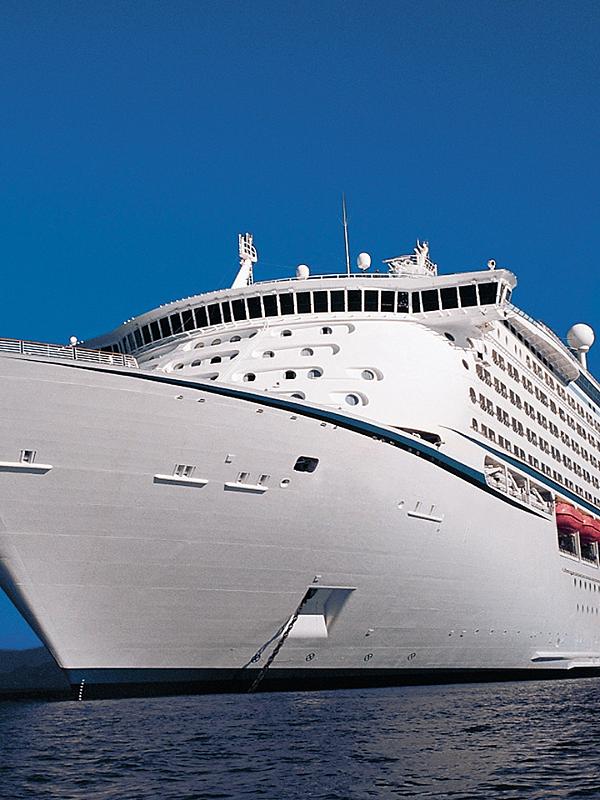The photograph captures a medium-sized, predominantly white cruise ship with blue detailing, anchored against a backdrop of a clear, dark blue sky and slightly moving dark water. The image, focused primarily on the front and part of the middle of the ship, showcases multiple levels with an array of black windows towards the upper deck, which likely include around 20 windows near the captain's area. Prominent on the right side of the ship are red lifeboats and staterooms with balconies. The ship features various antennas and GPS equipment atop, along with a large sphere-like structure and visible anchor chains at the forefront. The ship appears empty as there are no people visible on the deck, adding to the serene yet imposing presence of the vessel.